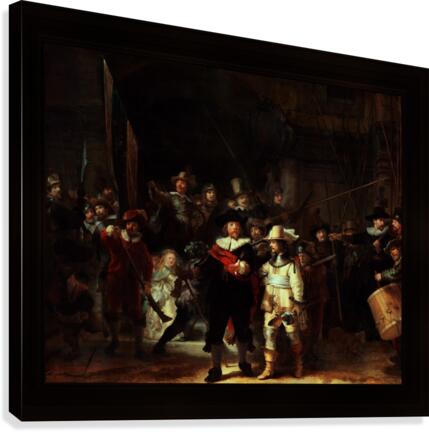The painting depicted is a classical and expertly crafted work, likely reminiscent of Rembrandt's style with its masterful interplay of light and shadow, marked by a predominantly dark palette of black, brown, white, and red hues. It is set within a solid black rectangular frame and viewed at a slight angle, with the right side tilted further away from the viewer. The scene captures a historical or Renaissance atmosphere with numerous figures dressed in intricate medieval garb, complete with hats and white collars, suggestive of social interaction. Central to the composition are two prominent men in the foreground, one with a dark beard and wide-brimmed hat, whose postures suggest significance and leadership. Around them, a crowd appears to be intently observing their actions, creating a sense of narrative tension. Additionally, a figure on the far right stands out, holding either a wooden drum or barrel, adding to the overall dynamic. The background is notably dark, which heightens the contrast and emphasizes the illuminated figures, drawing attention to their detailed expressions and attire. Overall, the painting radiates a rich, retro-classical aura that showcases skilled artistry and a deep, immersive historical ambiance.